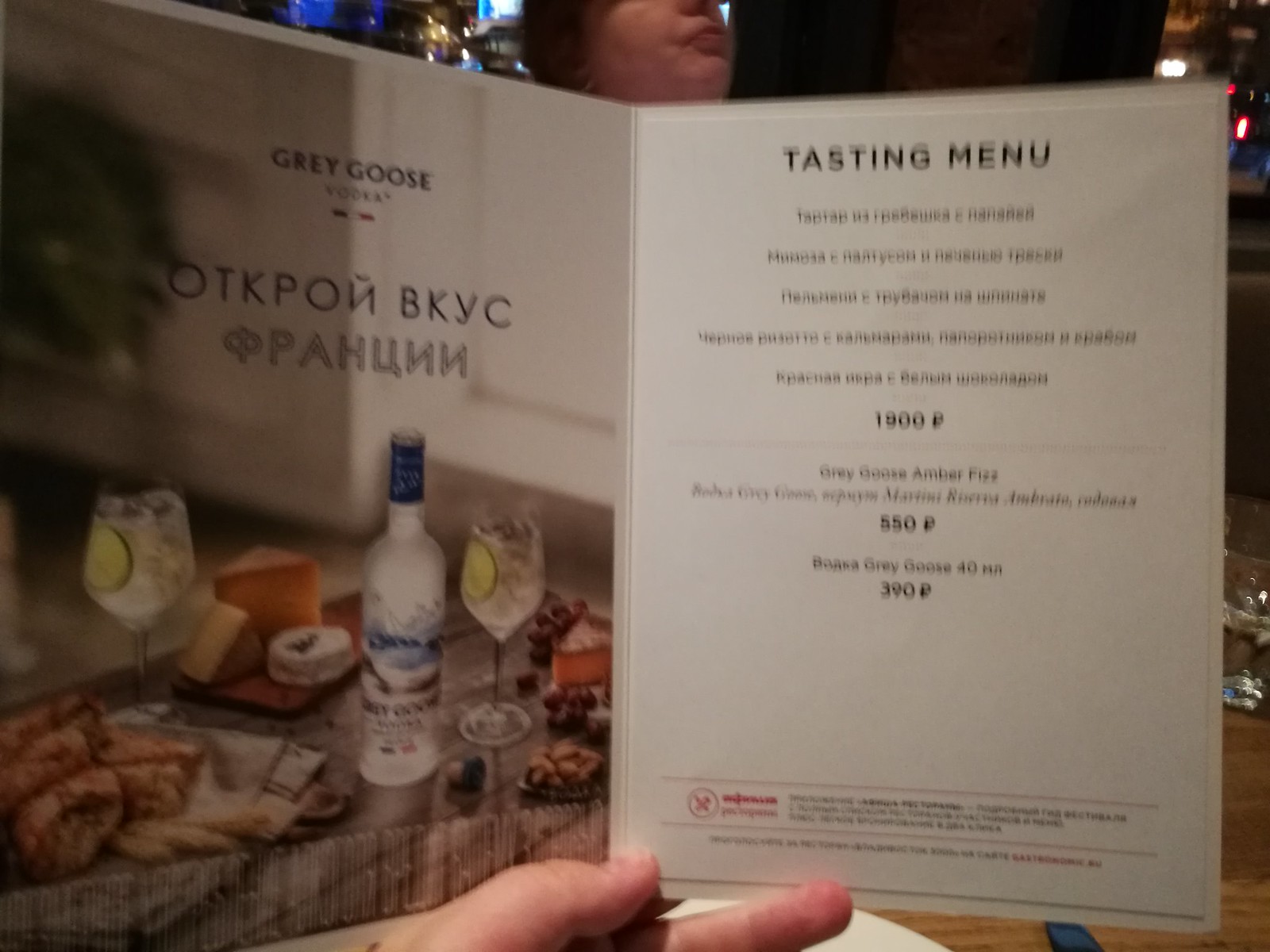In this vibrant color snapshot taken inside a lively restaurant, we see an intriguing blend of elements and details that capture the essence of the setting. The photo prominently features someone's left hand, their thumb and pointer finger gently resting on what appears to be a white plate, accompanied by a piece of silverware at the bottom center of the image. Above the hand, a folded menu commands attention, likely being held by another person across the table.

The intricacies of the scene continue with a cropped view of a woman’s chubby face at the top middle section of the photo. Her facial features include her mouth, nose, ear, cheek, and chin, but her eyes are out of the frame, adding an air of mystery. Surrounding her head, particularly to the left, are sparkling blue lights, potentially indicating an illuminated bar, while more lights embellish the right side of the background.

The right portion of the image showcases a wood-toned tabletop adorned with glassware, further enriching the restaurant ambiance. The focal point, however, is the elaborately detailed menu. On the left side of the open menu, an ad for Grey Goose Vodka draws the eye with its Cyrillic or possibly Ukrainian text. The ad features an enticing illustration of a Grey Goose Vodka bottle, accompanied by two stemmed glasses filled with a clear liquid, likely vodka with lime. This presentation sits on a tray brimming with a gourmet cheese board that includes types such as brie or camembert, and larger wedges of fancier cheeses perhaps like cheddar. The tray is complemented by a basket of assorted breads, grapes, olives, and other cheeses, creating a visually appetizing display.

On the right side of the menu, the text “tasting menu” is visible in white. However, due to the image's out-of-focus nature, the smaller text below "tasting menu" remains unreadable. There is a mention of what appears to be “1900” followed by a mysterious symbol that is indistinct, hinting at pricing or further descriptions that elude readability.

This snapshot intricately captures the moment and provides a feast for the senses, emphasizing the rich, detailed surroundings of a dining experience.